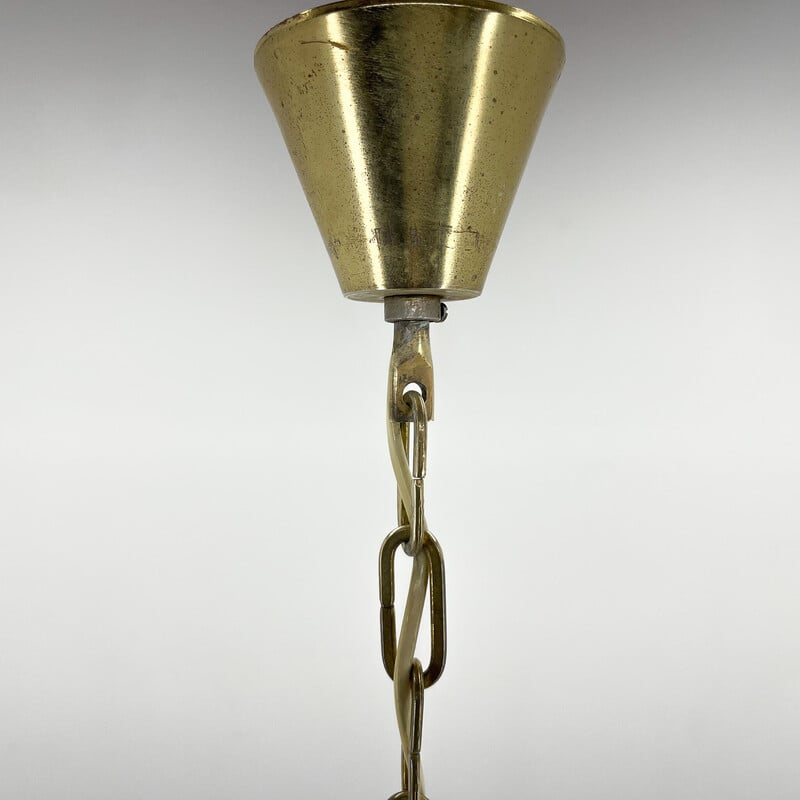This close-up image captures an inverted, tarnished gold bell-shaped object, centrally positioned within a wide vertical rectangle against a light gray background. The bell's cylindrical shape gradually widens towards what would traditionally be the lower end, but appears at the top due to its upside-down orientation. Its gold surface shows signs of wear, with visible brown spots and lines. At the bottom of the bell, a silver round screw is prominently attached. Suspended from this screw is a chain of interconnected links, which are rectangular with curved corners and slightly open edges, allowing them to hook together. The chain, along with some attached pipes, exhibits a dull brown or tarnished gold color. Winding through the chain's links is a light cream-colored wire, suggesting this assembly could be part of an old hanging lamp or measuring device, with the wire potentially serving as an electrical conduit.